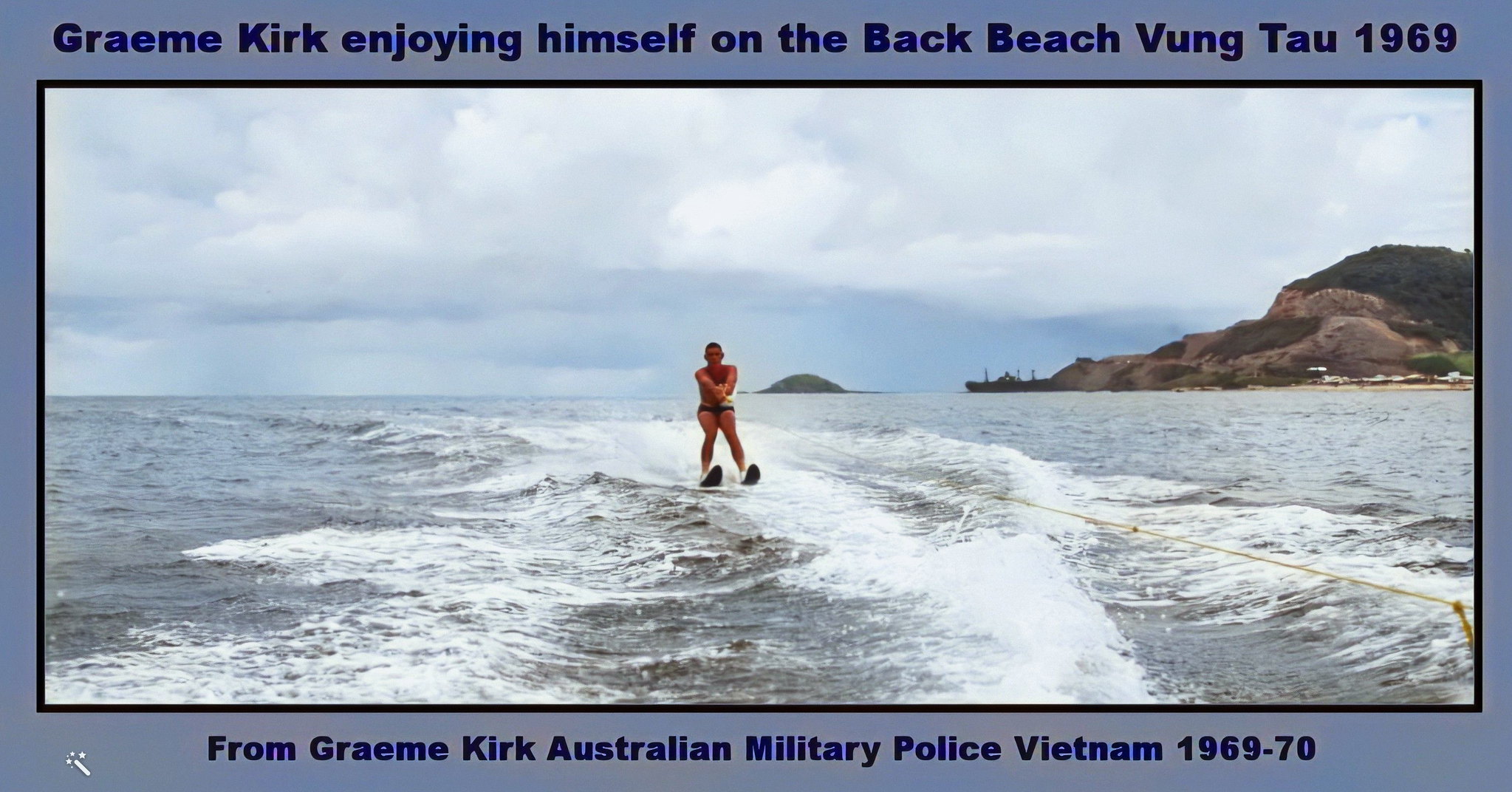In this detailed image, we see a man, Graham Kirk, water skiing against a backdrop of a rocky shoreline and an overcast sky. He is clad in tight, small, black shorts and is being pulled by a yellow rope, which stretches from his grip down to the bottom right-hand side of the frame, presumably connected to an unseen boat. The photograph captures the wake and white spray created by the boat, adding a dynamic element to the water in the foreground. The rectangular image is digitally framed with a gray-blue border, within which navy blue text at the top states, “Graham Kirk enjoying himself on the back beach, Vung Tau, 1969.” Additional text at the bottom reads, “From Graham Kirk, Australian Military Police, Vietnam, 1969-70.” The serene yet active scene, set under a mostly cloudy sky, with rocky hills visible in the upper right corner, paints a vivid picture of Graham Kirk’s moment of enjoyment in Vung Tau during that era.